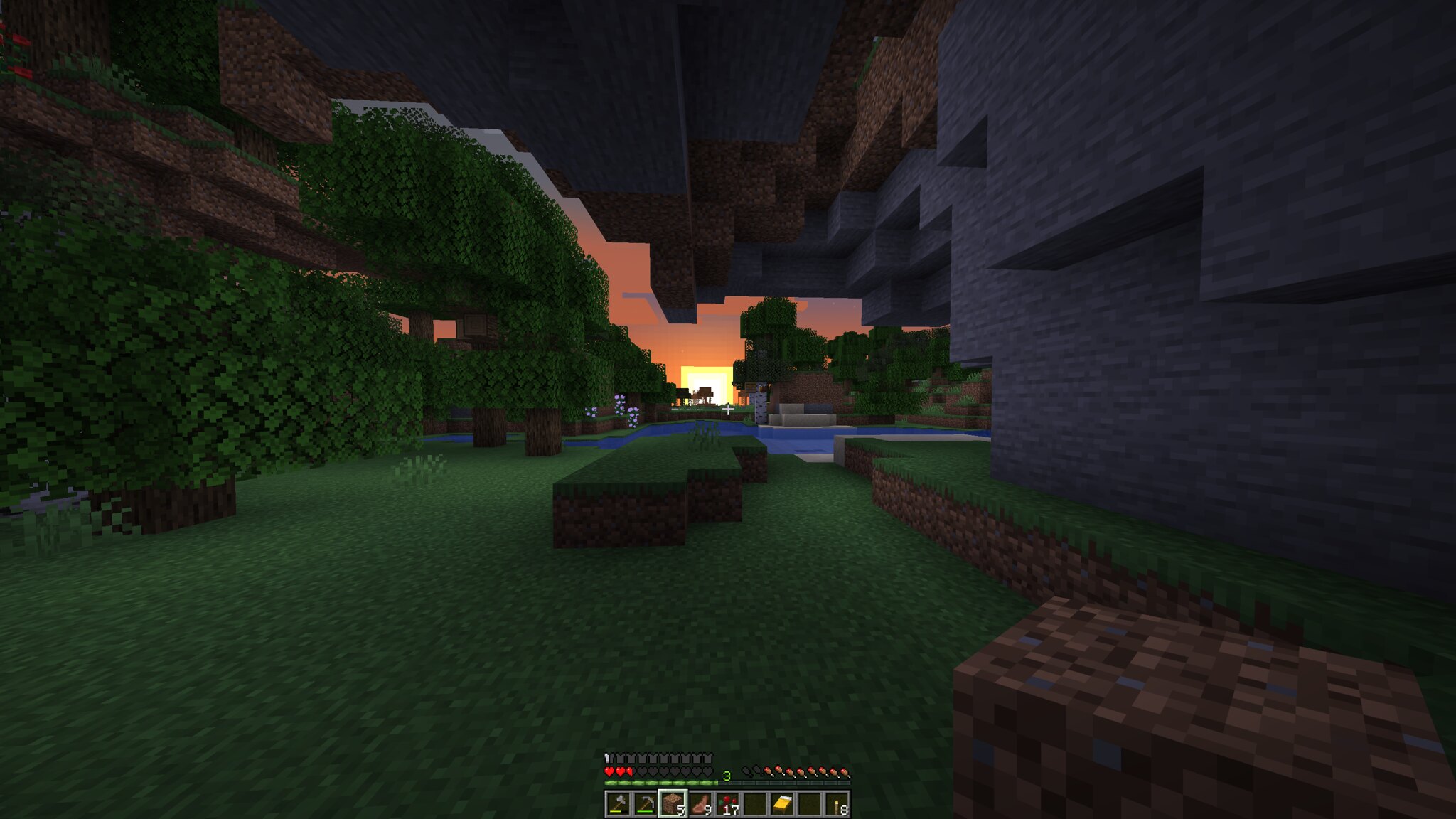The image showcases a vibrant video game scene displayed on a screen. The ground is covered in lush, neatly trimmed green grass, evoking the appearance of a well-maintained lawn. Along the sides, there is a striking gray brick building, constructed in a 3D style that gives the structure a dynamic, popping effect, making it feel as though it’s coming off the screen. In the foreground, there’s a multicolored box that appears to be made for sitting, featuring a palette of different brown shades, blue, and light brown. To the left side of the image, you can observe meticulously landscaped and manicured block trees, complete with a full canopy of leaves, adding to the scene’s rich, immersive detail.